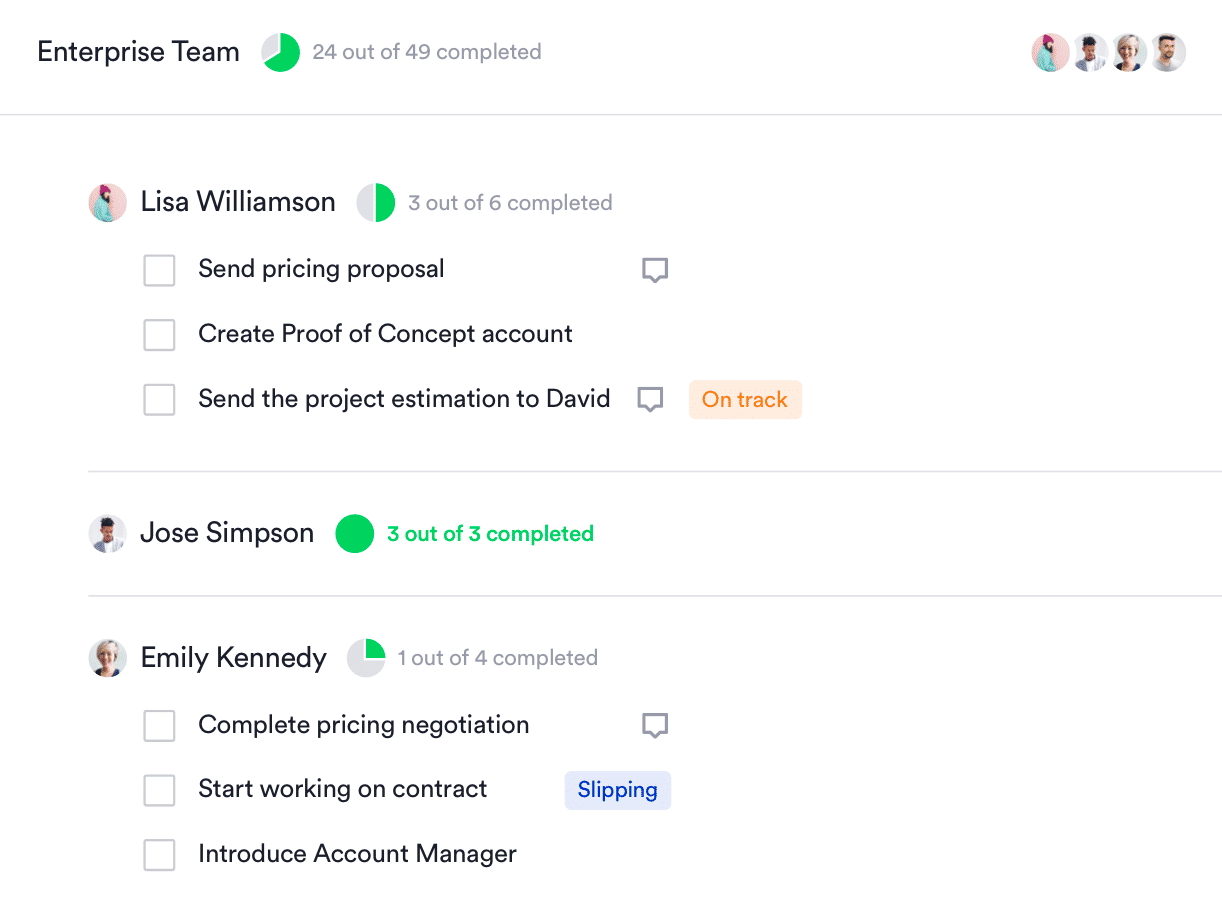A screenshot of a website featuring a clean white background. At the top right corner, there are three small profile pictures. The first profile picture shows a lady wearing a pink hat and a green shirt, looking sideways. Next to her is a black man in a light purple shirt. The third profile picture is of a woman with a short blonde haircut, and the fourth is of a man with dark hair. 

On the far left side, the text reads "Enterprise Team" with a symbol indicating "24 out of 49 completed." Below this section, the profile details begin with "Lisa Williamson," featuring the profile picture of the woman in the pink hat. A progress indicator shows "3 out of 6 completed." Adjacent to this, there are three checkboxes labeled:
1. Send pricing proposal
2. Create proof of concept account
3. Send the project estimation to David.

Each checkbox is followed by a small orange rectangular box that says "on track."

Following this, there is a section for "Jose Simpson," with his profile picture showing a man with dark hair. His progress indicator shows "3 out of 3 completed," marked with a green circle.

Lastly, the entry for "Emily Kennedy" is displayed, featuring the profile picture of the woman with short blonde hair. Her progress indicator shows "1 out of 4 completed." Underneath her name, the action items listed are:
1. Complete pricing negotiation
2. Start working on contract
3. Introduce account manager.